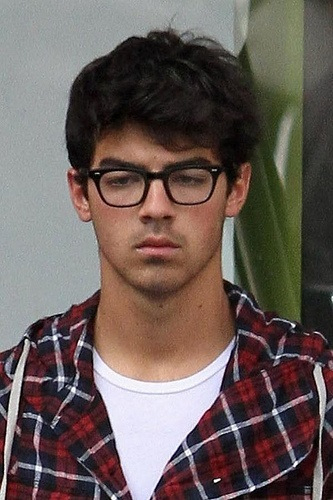This photograph captures a contemplative young man with a serious expression, his mouth closed, and a shadow of a mustache and beard. He has thick, wavy, fluffy dark brown hair that is short and layered, with strands falling over his forehead while the sides are clean cut. His thick, arched black eyebrows frame his face, which narrows down to an upside-down triangular shape with a narrow chin. Adorning his face are black-rimmed glasses with thicker, plastic-looking frames. His attire includes a white T-shirt beneath a red and black plaid jacket adorned with white stripes and two white hoodie ties emerging from the front. He appears to be leaning his head and left shoulder against an olive green-colored door or wall section, while the background primarily consists of a grayish or white wall, emphasizing the focused, introspective mood conveyed by his downward gaze.